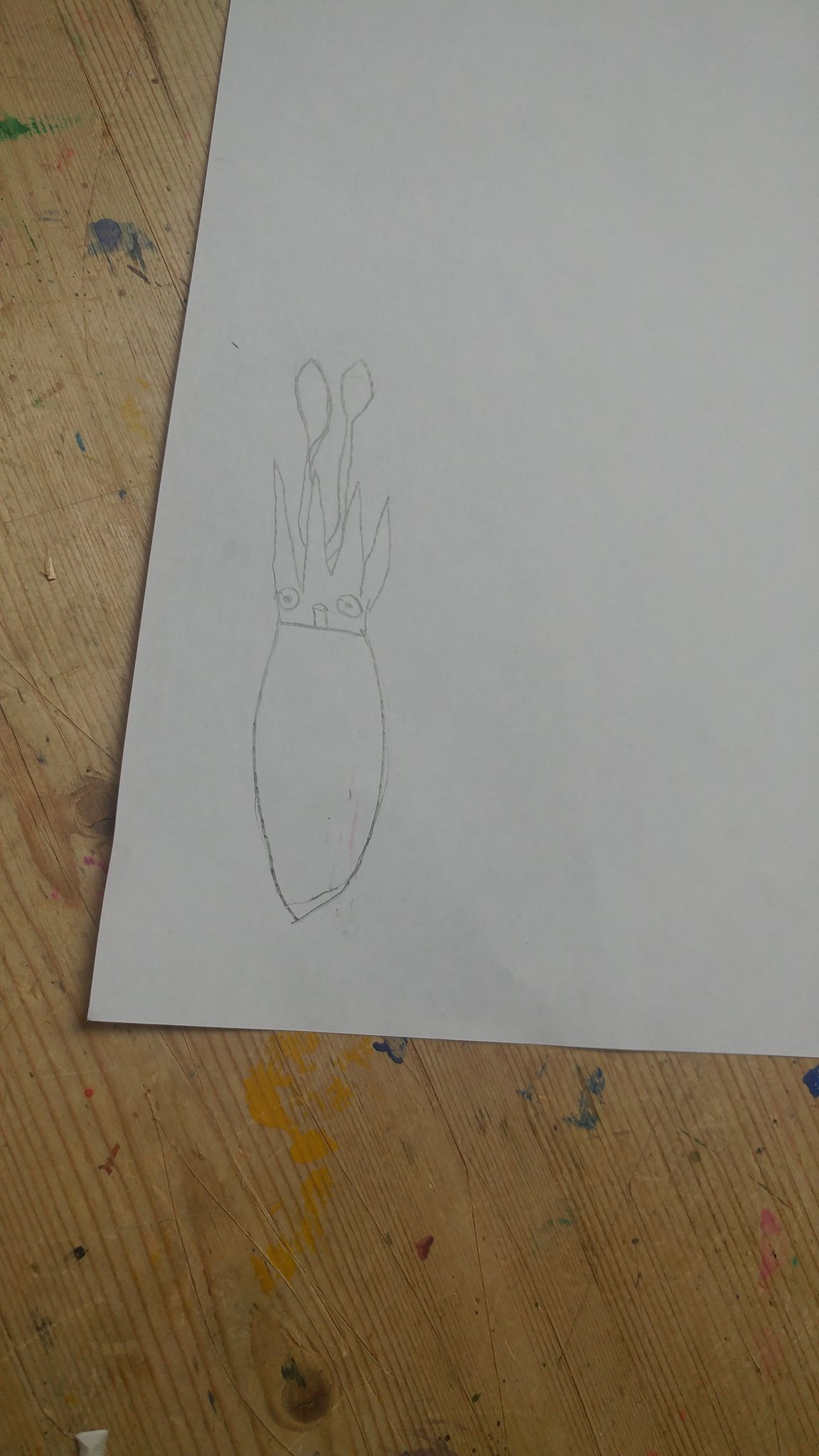The image features a detailed pencil drawing on the bottom left corner of a plain white sheet of paper. The focal point of the artwork is an oval-shaped creature with a flat top, resembling a cartoonish squid. The creature has two large, round eyes with black pupils and a small square nose. Its head is adorned with what appears to be flame-like spikes or plant leaves, and two spoon-shaped antennas extend from its head, each with a thin stem and a rounded, oval-shaped top. The mouth is an upside-down U shape, adding to its whimsical appearance. The sheet of paper itself shows faint wrinkle lines and occupies most of the image. 

The background reveals a worn wooden table, which shows signs of wear and tear, including scratches, cuts that suggest the use of an X-Acto blade, and various paint, pencil, and pen marks. The table adds to the rustic, artistic environment where this doodle was created. In the bottom left corner of the image, there's also a small, squarish piece of white plastic, partially visible.